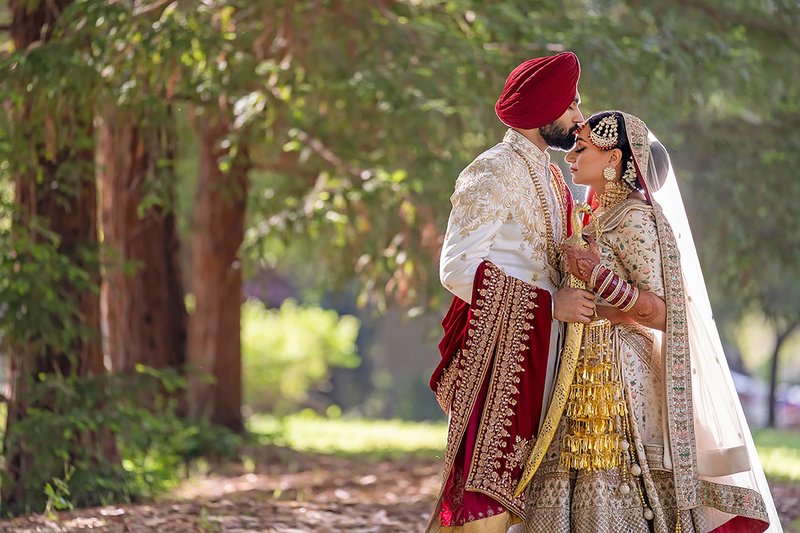In this horizontal image, an Indian couple stands on the right side of the frame in front of a walkway, framed by a backdrop of trees with brown trunks and green leaves. The couple appears to be dressed for their wedding day, wearing intricate and ornate traditional attire. The man, positioned on the left, is kissing the woman's forehead. He is adorned in a white long-sleeved shirt embellished with gold decorative elements and a long necklace. He wears a red turban and has a deep red and gold sash draped over his forearm, back, and shoulder. The woman, standing on the right, wears an elaborate patterned wedding dress featuring a white floral motif with gold accents. Her hair is styled in a bun, covered by a sheer long veil. She is adorned from head to toe with an array of jewelry, including large earrings and arm pieces. Both of them are holding a ceremonial gold sword, evoking the image of a royal couple. They stand surrounded by nature, under a canopy of trees that add to the serene and picturesque atmosphere.